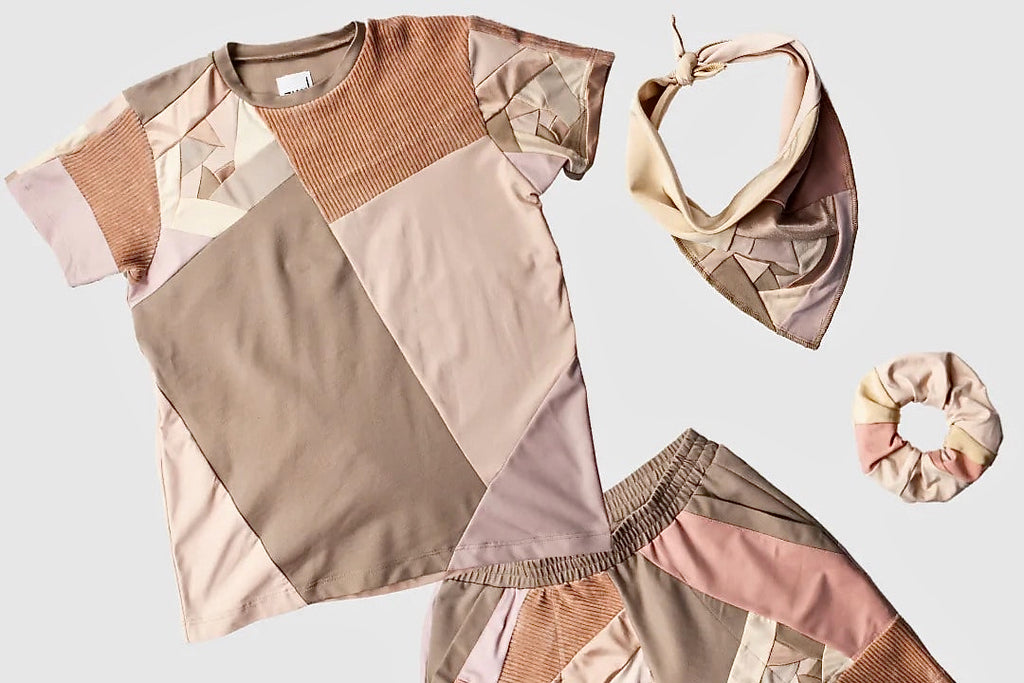This is a color photograph of a unique and eclectic women's outfit set, laid out on a white surface and photographed from above, reminiscent of a stylish catalog or Pinterest layout. The ensemble includes a short-sleeved t-shirt, a pair of shorts, a bandana, and a hair scrunchie. The t-shirt and shorts are crafted from various patches of neutral tones, including shades of brown, beige, and gray, giving them a rag quilt appearance with no symmetrical design—each piece of fabric is randomly sewn together. The shorts feature an elastic waistband for added comfort. The bandana, tied around the neck, and the scrunchie, lying nearby, coordinate perfectly in matching patterns and hues, completing the outfit. Despite the patchwork design, the overall look is cohesively coordinated, combining the distinctive colors and fabrics seamlessly.